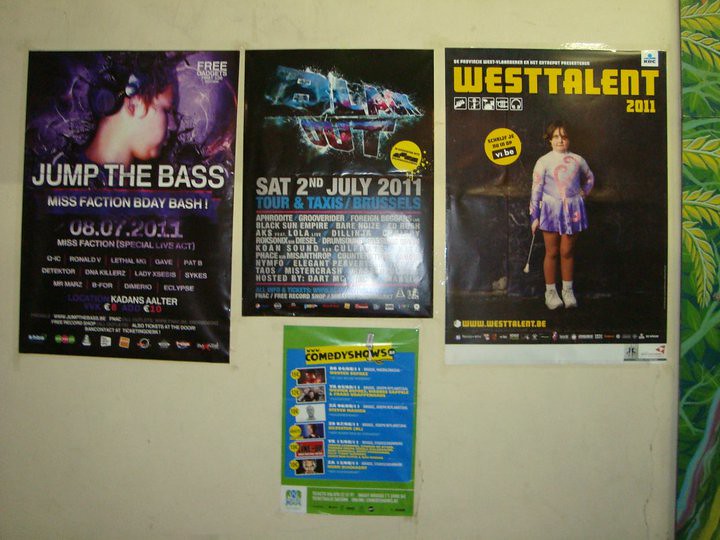The image captures a white wall with a touch of jungle-themed wallpaper on the right edge. Four posters, affixed with scotch tape, advertise various 2011 events. The top left poster features a dark purple background with white text promoting "Jump the Base, Misfaction Birthday Bash" with a profile view of a person looking right. The top center poster, smaller in size, uses white outlined, Star Wars-style lettering on black, announcing "Blackout" for Saturday, 2nd of July, 2011, at Tour & Taxis in Brussels. The top right poster, resembling a magazine cover, displays a chubby little girl in a purple and white majorette costume holding a baton, with "West Talent 2011" in yellow text at the top. The bottom poster is green and white, with several small images on the left side and a yellow rectangle with black text that reads, "The Comedy Shows."